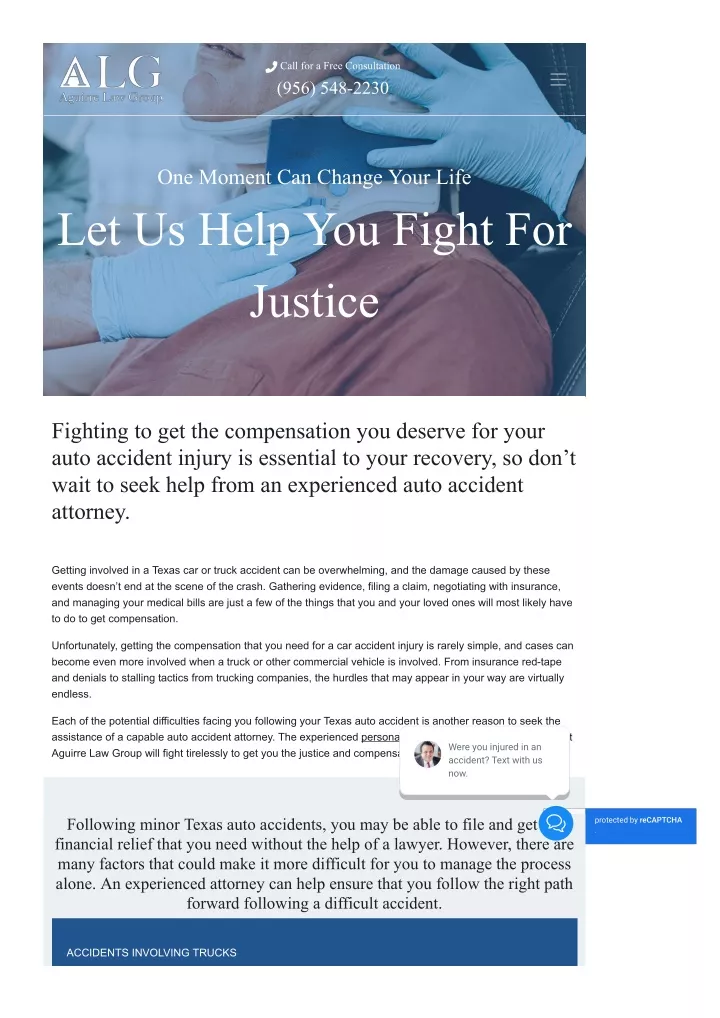A phone screenshot from ALG's website shows a header promoting a free consultation with the contact number 956-548-2230. Below, the tagline reads, "One moment can change your life, let us help you fight for justice".

The background image features a man in a reddish-orange t-shirt being fitted with a neck brace by two individuals. This visual underscores the urgency and seriousness of auto accident injuries.

The following text emphasizes the importance of securing compensation for auto accident injuries, describing it as essential to recovery. It advises not to delay seeking help from an experienced auto accident attorney, noting the complexity of car and truck accident cases in Texas. The text outlines the various challenges victims face, including gathering evidence, filing claims, negotiating with insurance, and managing medical bills. It highlights the intricate nature of obtaining fair compensation, especially when commercial vehicles are involved, pointing out issues like insurance red tape, denials, and stalling tactics from trucking companies.

A partially obscured paragraph suggests additional information blocked by a text tab, followed by a lighter gray section containing more text. The comprehensive depiction stresses the relentless obstacles in the pursuit of justice and the need for expert legal assistance.